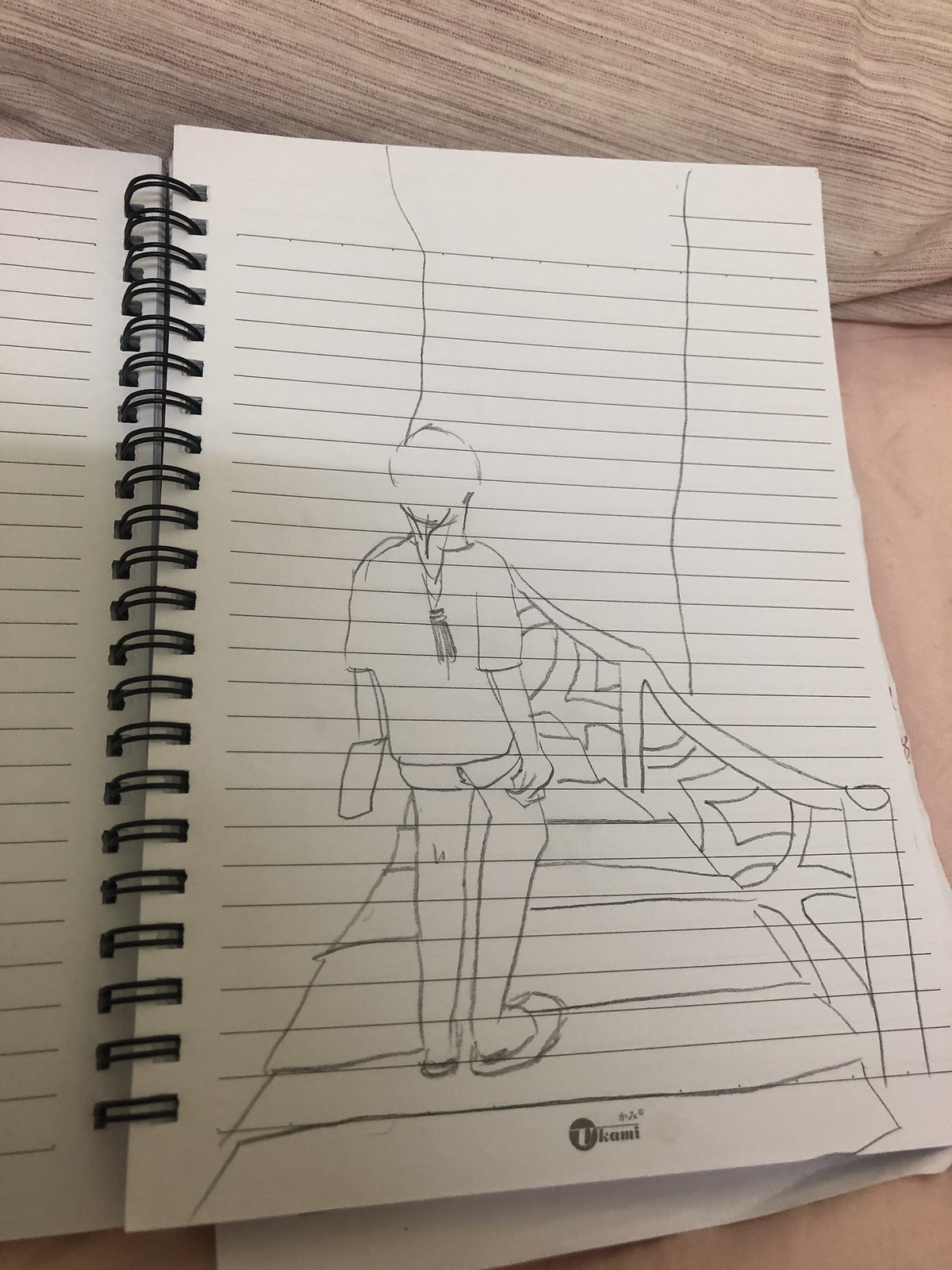This image captures a spiral notebook with black metal spirals, open to a single lined page with light blue, evenly spaced lines. On the right-hand page, there's a rudimentary pencil drawing of a person viewed from the back, walking on a wooden bridge. The person, possibly female due to the long hair styled in a ponytail or braid, is depicted as wearing a short-sleeved top, short shorts, and slip-on sandals. While the right hand of the figure is drawn with some detail, the left hand appears to be a simple square. The bridge features diamond-patterned cutouts in its intricate railing to the right of the figure. Above the figure are two horizontal lines that span across both pages. The scene is set indoors, with a striped pillow case in various shades of gray and off-white visible at the top left of the photo, and an off-white blanket partially in view at the bottom corners.